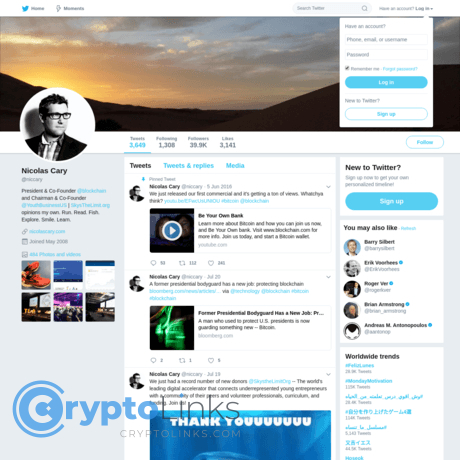The image showcases a Twitter page with a watermark in blue on the bottom left corner that reads "Cryptolinks." The page belongs to Nicholas Carey, featuring his profile avatar on the left side where he's seen wearing glasses. The header image at the top of the page depicts a scenic landscape with a captivating sunset in orange hues and grey clouds against a black foreground.

At the top right of the interface, there is a search icon and a search bar. Below it, login fields invite users to enter their phone, email, or username alongside password information. A "Remember me" checkbox, a "Forgot password" link, and a prominent "Login" button are also visible. For newcomers, there's a "New to Twitter?" prompt followed by a blue "Sign up" button.

The navigation tabs at the top of Nicholas Carey's Twitter page include "Tweets," "Tweets & Replies," and "Media," with the "Tweets" tab currently highlighted in blue. The stats reveal 3,749 tweets, 1,308 people followed, and 39.9k followers, with 3,941 listed under "Next." A "Follow" button is present on the right side.

An invitation to sign up for Twitter appears on the right, with some suggested connections, although the text is slightly blurry and small. At the bottom, a white "Thank you" message is displayed, and a grey-colored link to "cryptolinks.com" is provided.